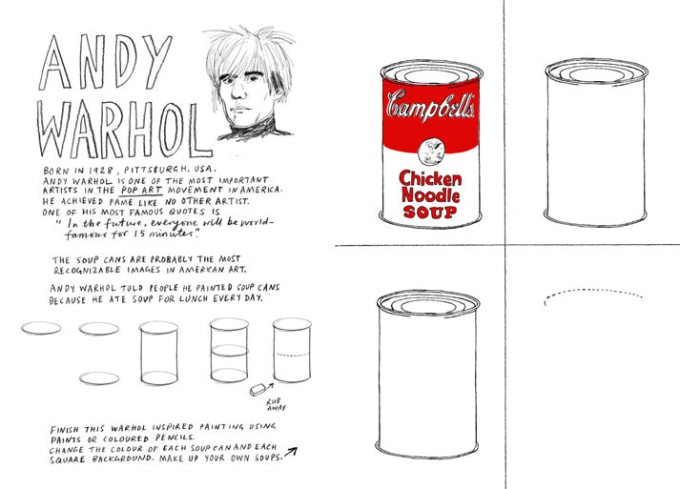This detailed illustration serves as a tribute to Andy Warhol, focusing on his iconic pop art Campbell's soup can. It features the handwritten name "Andy Warhol" in the top left corner, accompanied by a portrait of Warhol, identifiable by his shaggy hair and dark eyebrows. Below his name, a textual biography states, "Born in 1928, Pittsburgh, USA, Andy Warhol is one of the most important artists in the pop art movement in America. He achieved fame like no other artist. One of his most famous quotes is, 'In the future, everyone will be famous for 15 minutes.'"

The main part of the illustration teaches viewers how to draw the Campbell's chicken noodle soup can in a step-by-step manner. There are partial sketches depicting the progressive stages of drawing the can, arranged in a grid format with four distinct stages. In the upper left of the grid, a fully colored red-and-white Campbell's chicken noodle soup can is prominently displayed, featuring "Campbell's" in white font on a red background and "chicken noodle soup" in red on a white background. Beside this can, the same can appears without its label, showcasing the traced outline. Further stages illustrate the drawing process, including a plain white can with black trim and a detailed top view.

The entire composition is set against a white background and is rendered in black-and-white with selective uses of red to highlight the soup can. This comprehensive visual guide not only celebrates Warhol's art but also underscores his influence and the enduring recognition of his work, especially his famous soup cans which he painted because he ate soup for lunch every day.